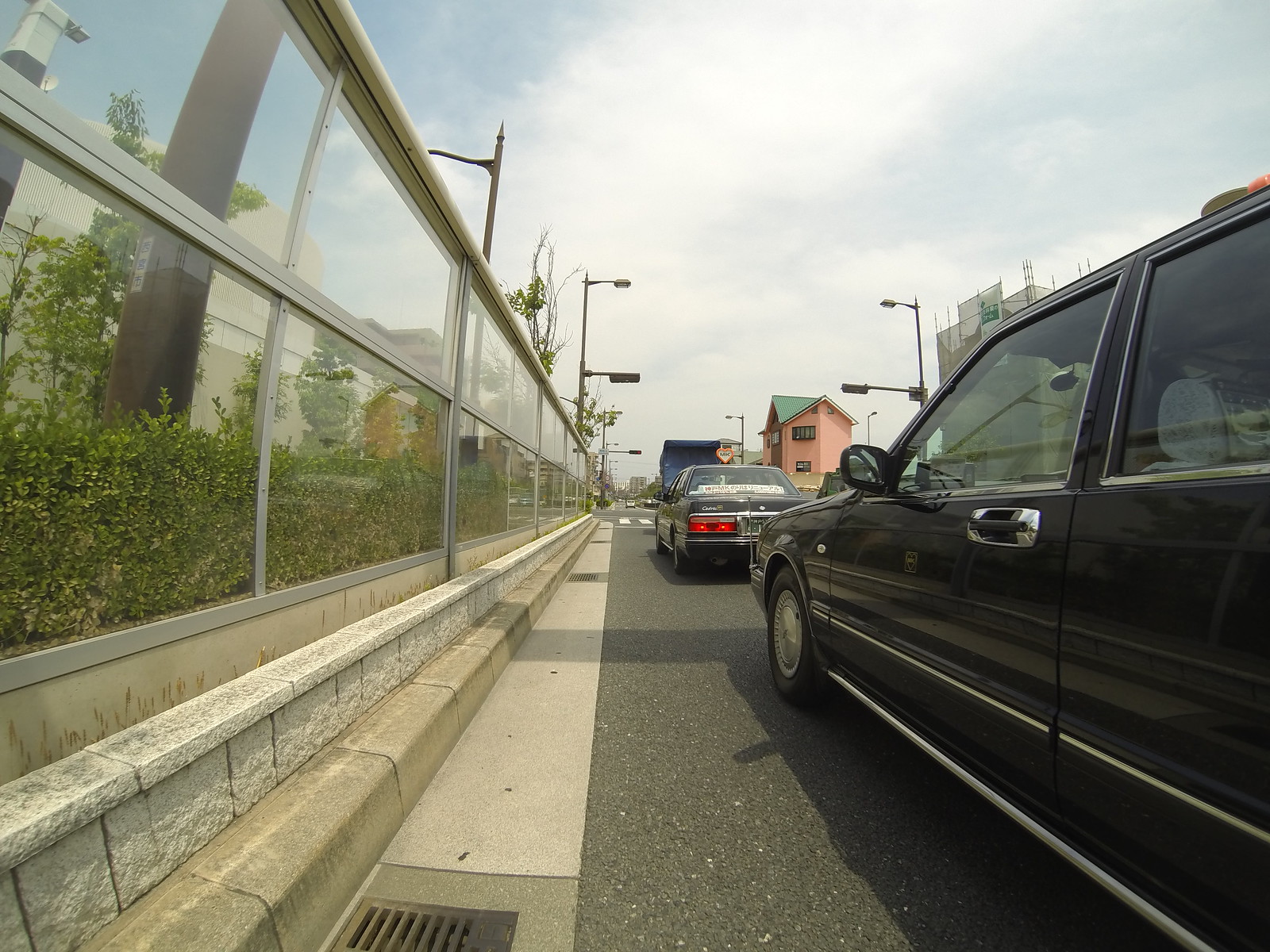The photograph features a bustling street captured from the perspective of the left lane. On the right side of the road, a line of cars and trucks, including a prominent black limousine with reflective windows and another black sedan, are neatly parked along the edge. The dark pavement transitions into a lighter gutter area featuring a sewer grate, followed by a distinctive curbing setup; a lower curbing section supports a white stone curb, above which glass or plexiglass panels are mounted in two rows separated by gray dividers, topped with a gray railing.

On the opposite side of these panels, patches of green plants flourish, leading up to a building on the left. The right side of the road boasts additional structures, including a peachy salmon-colored building with a greenish roof, likely two to three stories high. The street is lined with streetlights and adorned with some trees, further emphasizing its busy nature and significant traffic flow. Above the scene, a blue sky filled with patches of white clouds provides a serene backdrop, contrasting the hustle and bustle below.